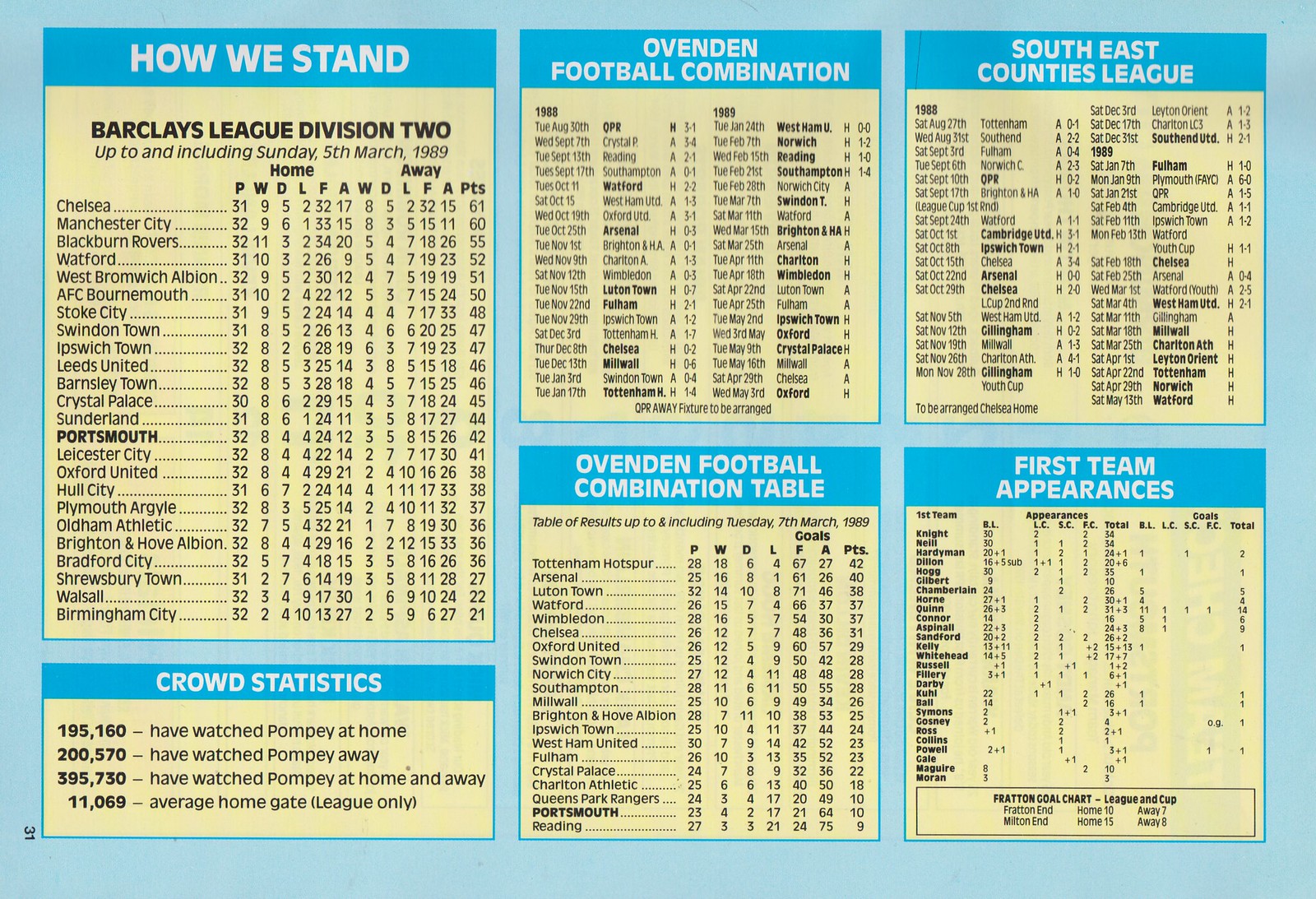This horizontally aligned rectangular poster features a light blue background and is filled with six distinct informational boxes. On the upper left-hand side, the largest box is titled "HOW WE STAND" in all caps with white letters. This section details the standings in the Barclays League Division Two up to and including Sunday, March 5th, 1989, listing various cities and summarizing home and away points in separate columns. Directly below this, a smaller box labeled "CROWD STATISTICS" presents the number of people who have watched Pompeii at home and away matches, along with the average home gate for league-only games.

To the right of these boxes are four smaller sections arranged in a two-by-two grid. The top-left box is titled "OVENDEN FOOTBALL COMBINATION" and includes information from the years 1988 and 1989. Adjacent to it, on the top-right, is another box labeled "SOUTHEAST COUNTIES LEAGUE," also featuring league statistics and scores. Directly beneath "Ovenden Football Combination" is the "OVENDEN FOOTBALL COMBINATION TABLE," which provides a detailed table of results, including cities, their goals, and points, up to and including March 1989. Finally, in the bottom-right corner, the "FIRST TEAM APPEARANCES" box lists names, appearances, and goals, although this section is in smaller print and slightly harder to read.

Each section header is set within a blue rectangle with white text, while the main body of these boxes features a light yellow background with black text, bordered in blue. This comprehensive poster, filled with intricate details, offers a thorough overview of football statistics, standings, and crowd data from the late 1980s.